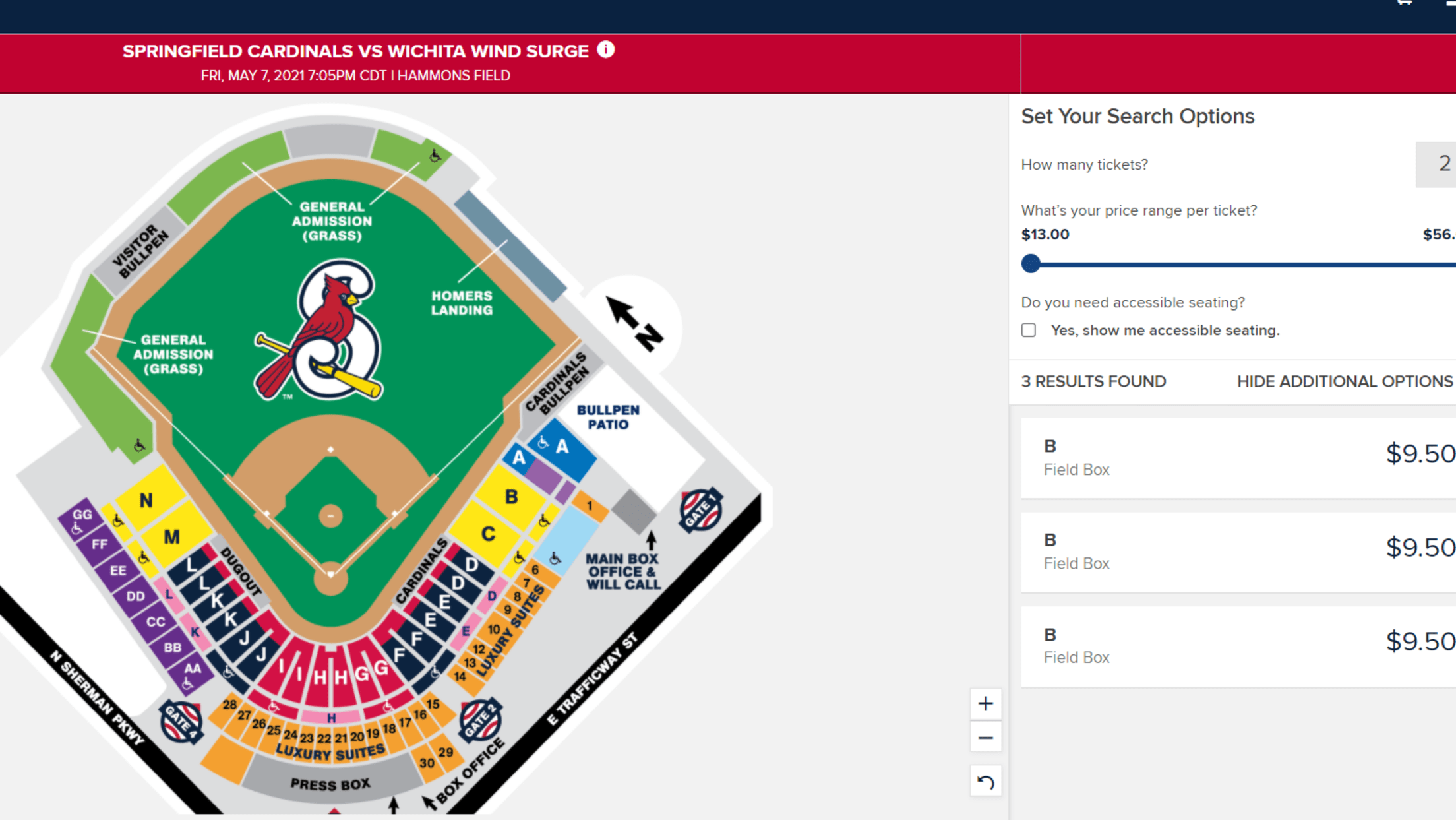This image features a detailed seating chart of a stadium for a baseball game between the Springfield Cardinals and the Wichita Wind Surge. The chart provides a comprehensive view of the field, depicted in vibrant green, as well as the entire stadium's seating arrangements. A key on the right side of the image allows users to set search options, including the number of tickets, from as little as two examples, and defines a price range per ticket from $13 to $56. 

The chart also includes an option for accessible seating, allowing users to specify if they need accommodations such as wheelchair accessibility. Based on the search criteria, three seating options are displayed, all located in the B section of the field box and priced at $9.50 each.

The visual representation of the stadium is colorful and informative, with a red cardinal symbol prominently displayed on the field. The seating areas are color-coded—purple, yellow, red, black, and pink—making it easy to identify various sections, including special areas like the press box and the bullpen patio. This practical layout helps first-time visitors choose their preferred seats based on proximity to different amenities and points of interest within the stadium.